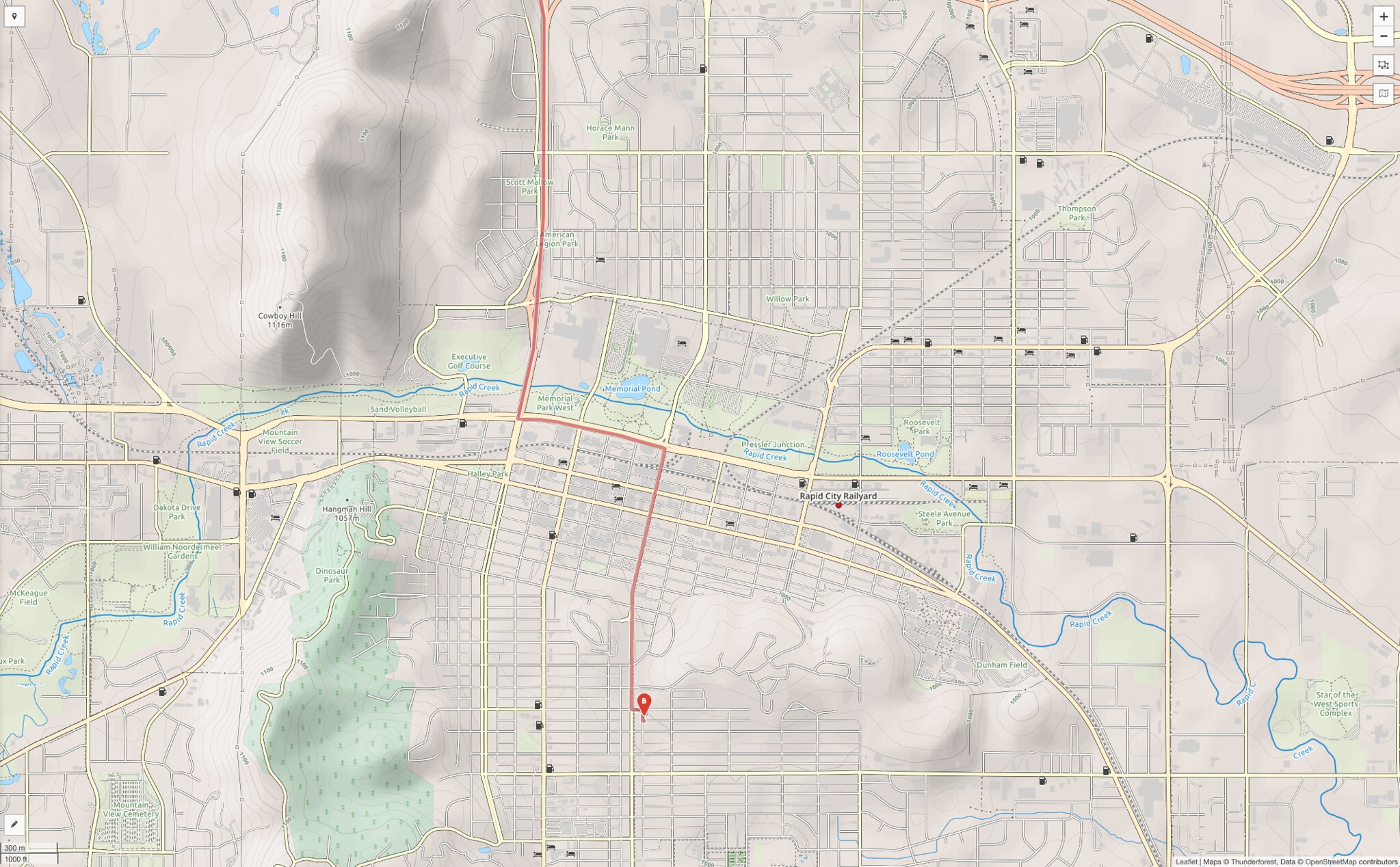The image is a detailed map, reminiscent of what you might see on a real estate website or during a navigation session. The map features an off-white background adorned with various dividing lines in dark gray, which likely denote different property boundaries or neighborhood divisions. These gray blocks probably signify houses or residential areas. Overlaid on these blocks are yellow lines and blue lines, which likely represent roads and waterways, respectively. 

Additionally, the map depicts various elongated areas of green and blue, suggesting parks, natural reserves, or bodies of water. There are also stretches of dark gray, possibly indicating industrial zones or undeveloped land. 

A prominent red line runs nearly down the center from the top of the image, veering sharply to the right halfway down and continuing further before ending in a location marker icon, likely indicating a destination. Overall, the map appears to illustrate a set of directions or a planned route to a particular place, providing a comprehensive view of the surrounding area as well.